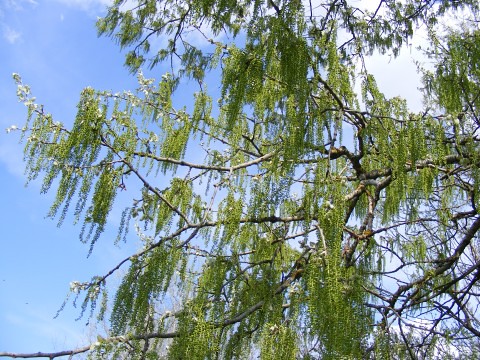An outdoor daytime shot captures a tree, likely a weeping willow, with its thin, brown branches and cascading green vines resembling a waterfall. The scene is bathed in sunlight, illuminating the upper right corner where the blue sky is dotted with wispy white clouds. Interspersed among the hanging vines are delicate flower buds, tinged in light purple or pink. The tree's dense network of branches occupies much of the image, especially more tangled at the bottom right, providing a stark contrast to the tranquil sky and the few clouds visible through the foliage.